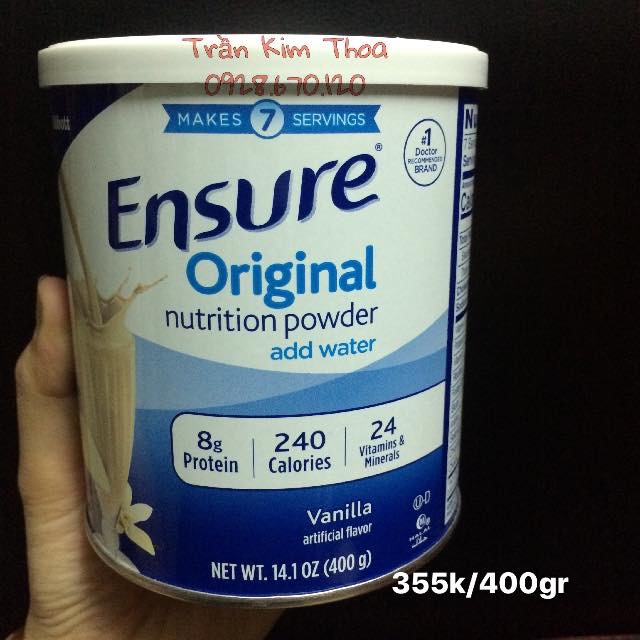A picture showcases a hand holding an Ensure Original Nutrition Protein Powder can. The hand, likely the person's left, is positioned with the thumb and the lower part of the palm visibly facing the viewer. The Ensure canister, predominantly occupying the image, is round with a metal base and a white lid. The packaging features various shades of blue, with "Ensure Original Nutrition Powder" displayed prominently. Beneath this, the words "Add Water" are inscribed. The design features two light blue bands at the bottom that gradually merge into darker hues. A white strip on the canister highlights nutritional information: "8 grams of protein, 240 calories, and 24 vitamins and minerals." Below this, it mentions the vanilla artificial flavor and the net weight of "14.1 ounces (400 grams)." To the right of the canister, an illustration shows the vanilla shake being poured into an old-fashioned soda fountain glass, enhancing the appeal. To the left, there's a barely visible sliver of the nutrition label. The background of the image is black, contrasting with the colorful details of the canister.